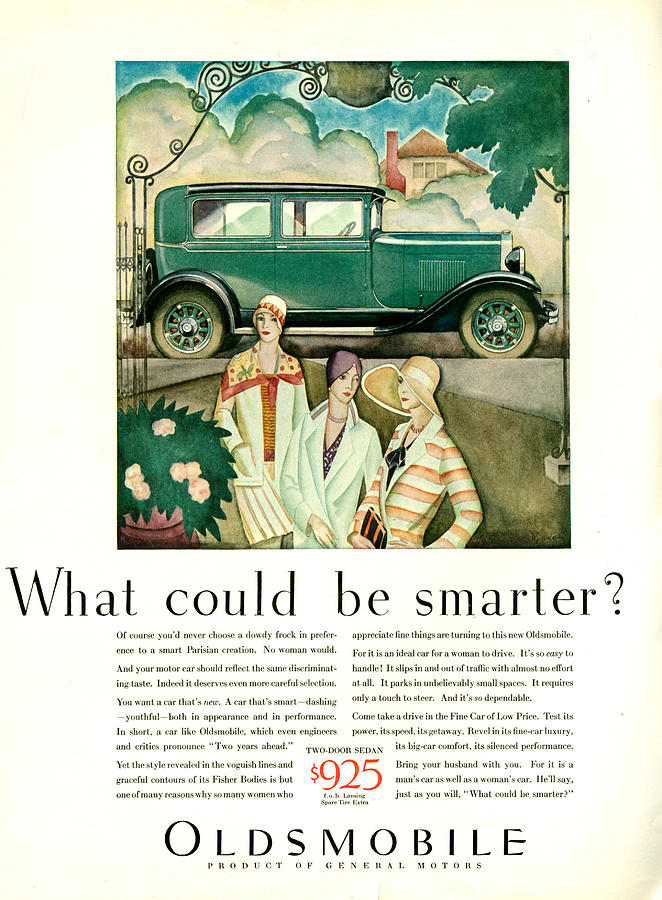The image is a vintage advertisement for an Oldsmobile, depicted as a detailed painting or drawing on a magazine page. The centerpiece of the illustration is a classic green Oldsmobile, with four rectangular windows and distinctive tires featuring a yellow outline and rims with green spokes. The setting includes a scenic background with a fancy house and a wrought iron gate, adding to the sophisticated ambiance.

In front of the car, three stylishly dressed women stand on a grassy area. The woman on the left wears a white cap and a light jacket accented with a yellow background over the shoulders and a red edge. The woman in the middle sports a purple headdress and a light blue coat, while the woman on the right is adorned with a yellow hat with a wide brim that nearly hides her face.

The top of the advertisement features the text "What could be smarter?" In the center, there is a bold mention of the price: "$925, two-door sedan." The advertisement emphasizes the car's appeal to women, highlighting its ease of handling and maneuverability in traffic and tight parking spaces. The bottom of the ad proudly states, "Oldsmobile, product of General Motors," all set against a slightly yellowed backdrop, suggesting vintage charm and nostalgia.

The colors used in the image range from various shades of green on the car to the diverse palette in the women's attire, including shades of white, purple, blue, yellow, and red. The overall presentation suggests an elegant and sophisticated life, captured in the timeless appeal of the Oldsmobile.